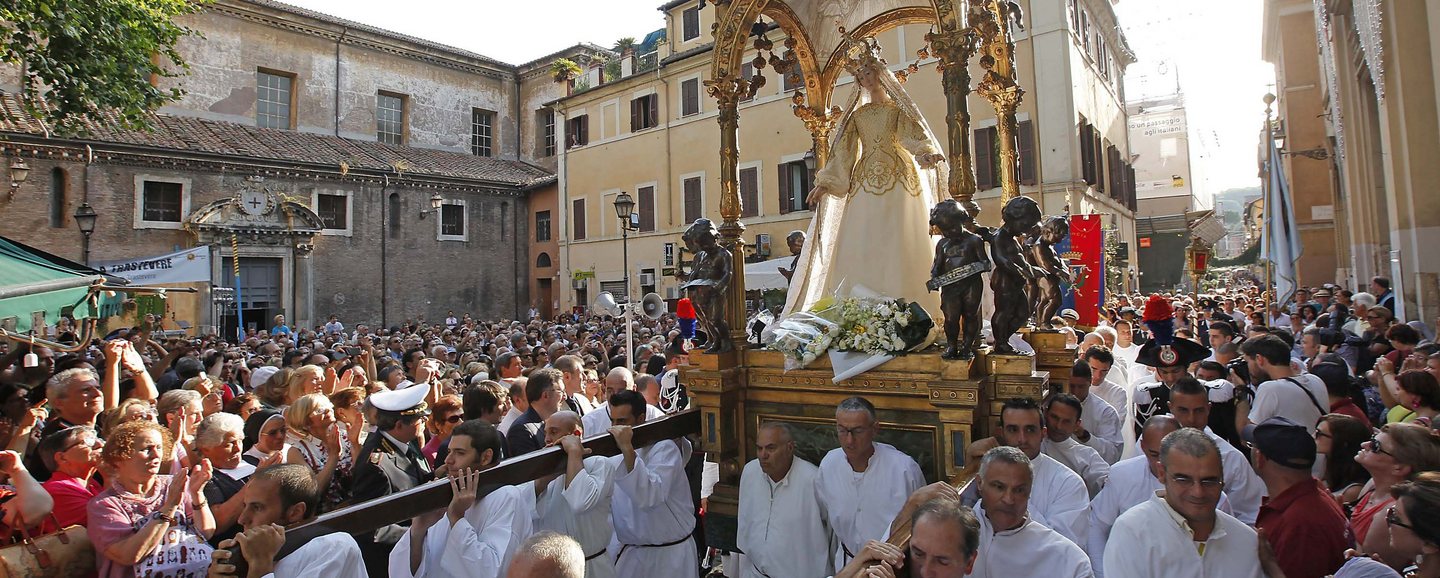This photograph captures a vibrant and densely attended religious procession in what appears to be a European, possibly Italian, town square, adorned with stucco-fronted stone buildings. Central to the image is an ornate, rococo-style float being carried by numerous men dressed in white tunics with black belts. The float itself is a wooden structure, lavishly decorated with cherubic statues and a canopy. At the heart of this elaborate platform stands a statue of a woman adorned in a long white gown with an overlay of gold on the upper half, a flowing white veil, and a gold crown. Her feet are surrounded by an array of flowers. The streets are thronged with townspeople standing shoulder-to-shoulder, engrossed in this grand and possibly Catholic spectacle. The detailed craftsmanship and decorative elements of the float, combined with the historical architecture of the town, evoke a sense of deep tradition and communal reverence.